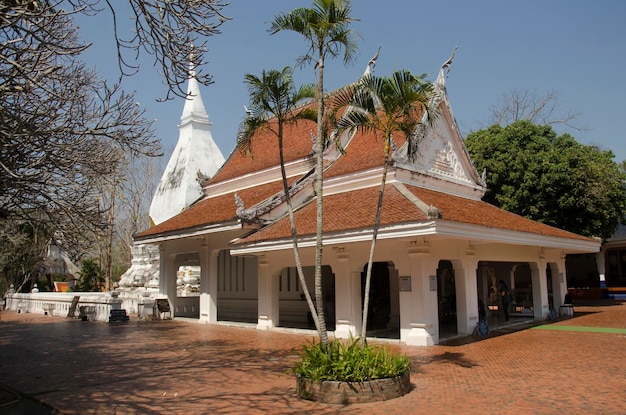The image showcases a bright and clear outdoor photograph of a striking Buddhist temple, or Wat, characterized by its distinctive architectural elements. This white temple features large columns around the first floor and is crowned with a roof made of reddish-brown clay-like shingles with ornate, curved ends. Small statues are positioned at the corners of the roof, adding to the temple's grandeur. 

In front of the temple, three slim trees grow within a small circular enclosure of grass, framed by the reddish-tinged tiled floor that surrounds the area. To the left of the temple stands a white pagoda-like tower, partially obscured by tree branches and protected by short white fences. The scene is bathed in natural light under a clear blue sky, adding to the image's vibrant and serene atmosphere.